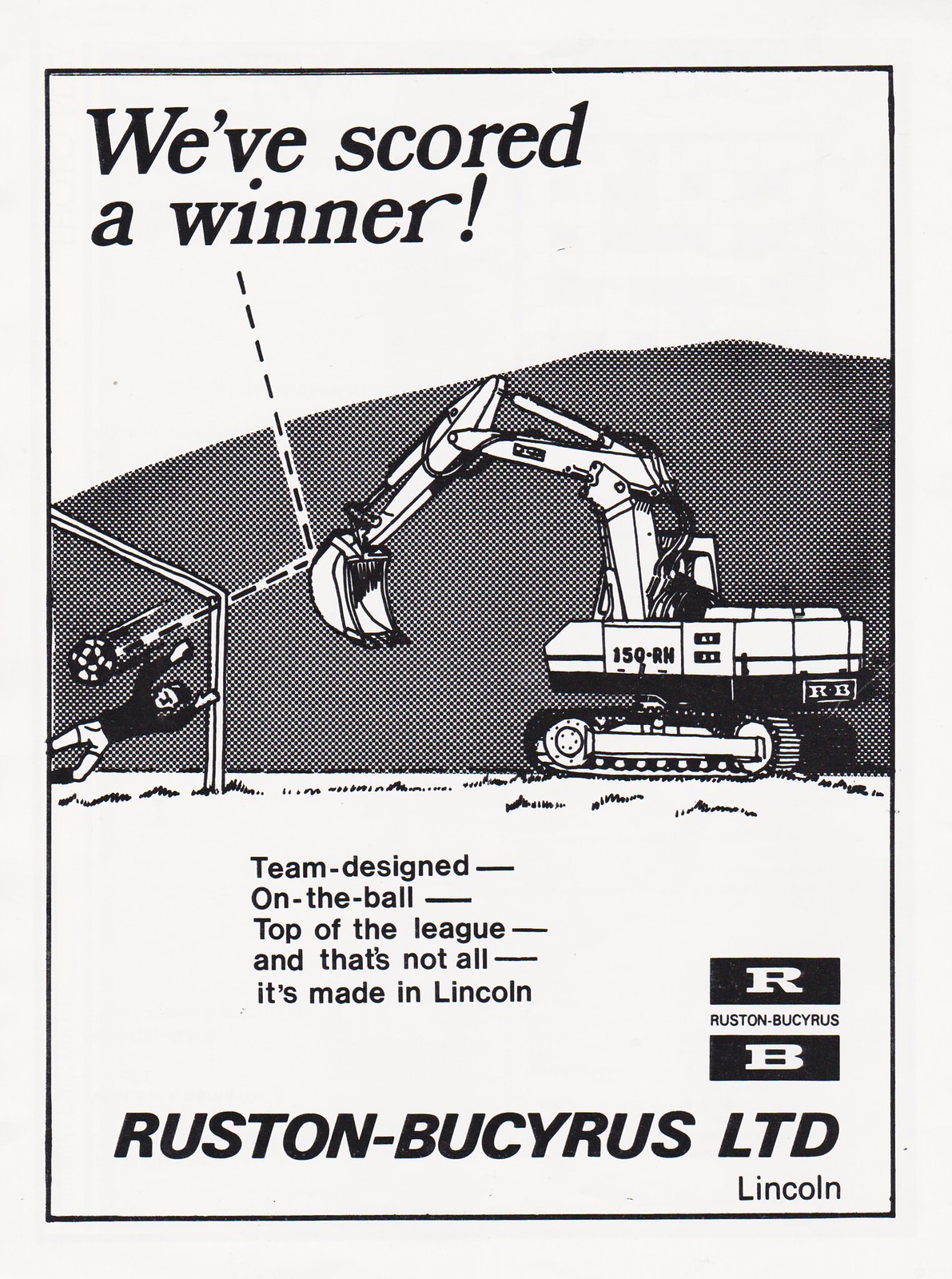This is a full-page advertisement most likely from a game day program or magazine, featuring a promotional message with a sports theme. The ad has a simple, clean design with black print on a white background, and it is framed by a thin black border. At the top of the page, bold text reads "We've scored a winner!" accompanied by a detailed hand-drawn illustration of an excavator identified as the 150-RH model. This heavy-duty machinery, equipped with roller treads, is depicted dynamically intercepting a soccer ball mid-air. 

The ball's trajectory is indicated by a dotted line that starts from the top, striking the scoop of the excavator, and directing it toward a goal. Against the left of the image, a soccer goalie is shown diving in an attempt to block the ball but is clearly outmatched by the excavator. Below the action-packed illustration, the text proudly declares "Team designed, on the ball, top of the league, and that's not all. It's made in Lincoln."

The bottom section of the advertisement further credits the manufacturer, with the names "Ruston Bucyrus Limited" and "Lincoln" prominently displayed. The company's logo features two distinctive boxes: one with a white "R" on a black background and another with a white "B" on a black background.